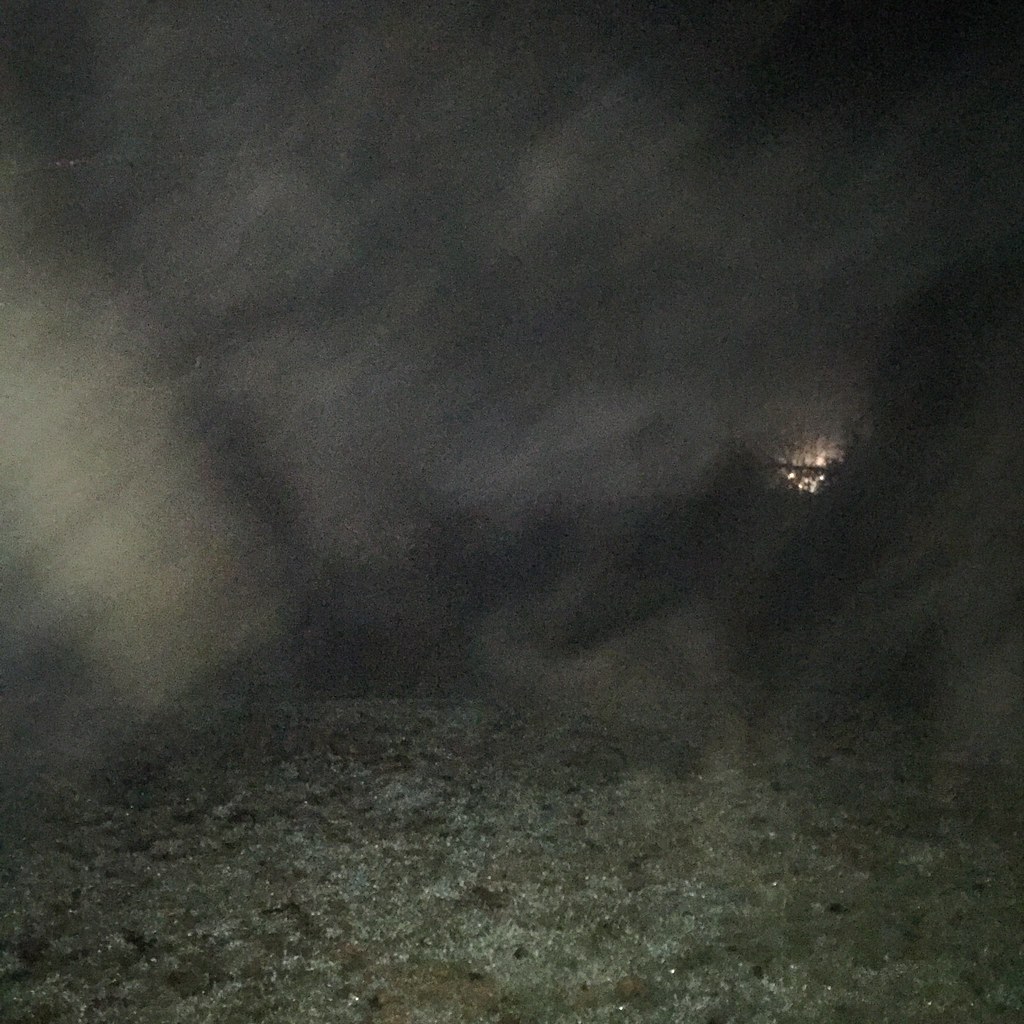This is an extremely blurry, mist-covered outdoor photograph that initially appears to be an abstract art piece due to its smeared and mottled texture. The foreground features a lumpy, gray surface that resembles a mix of sand, stones, and possibly weeds, though the exact details are indiscernible. Dark grays and browns dominate this area, with specks of black hinting at a stone texture. The horizon cuts across the image at a slant, above which lies a misty, foggy sky filled with dark gray and bluish tones interspersed with lighter gray or white mist. Among these smoky, misty shapes, some black and very dark silhouettes give an eerie impression, almost like ghostly figures. In the distant center of the image, a tiny, brighter spot of pale orange light suggests a small fire that must be substantial given the amount of smoke filling the scene. The distant glow also gives an illusion of lights nestled beneath or within a parallel line, possibly from a far-off fire or illuminated trees, adding to the overall spooky, supernatural ambiance of the photograph.